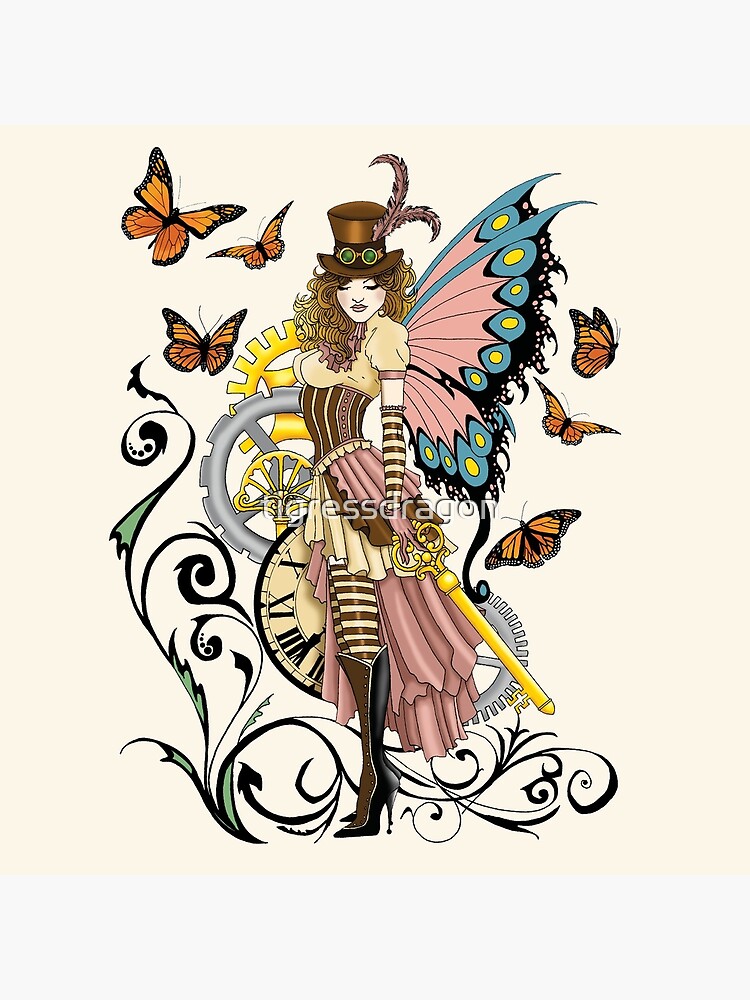This is an intricate artist's sketch of a woman dressed in an elaborate steampunk-themed outfit. She stands in profile, facing the left side of the image, but stares directly at the viewer. Atop her head rests a stovepipe hat adorned with goggles positioned above her forehead. Her attire features a detailed brown and white corset worn over a yellowish-white blouse, paired with a yellowish-whitish skirt. She wears striped leggings and knee-high, heavy leather or possibly metallic boots with very high heels.

Completing her fantastical look are butterfly wings, colored predominantly in pink with blue and black at the ends, adorned with yellow circles. She is holding an exotic key, suggesting a sense of mystery. Set in the midst of a steampunk-inspired background, she is surrounded by silver and gold gears, a clock with Roman numerals, and monarch butterflies. Vines climb amidst the gears and butterflies, adding to the intricate and whimsical scene. The background features a gradient from bluish white at the top and bottom to a peach or mauve hue in the middle, blending with green-yellow scrollwork and monarch butterflies throughout. A watermark spans the center, lightly obscuring some elements of this detailed composition.